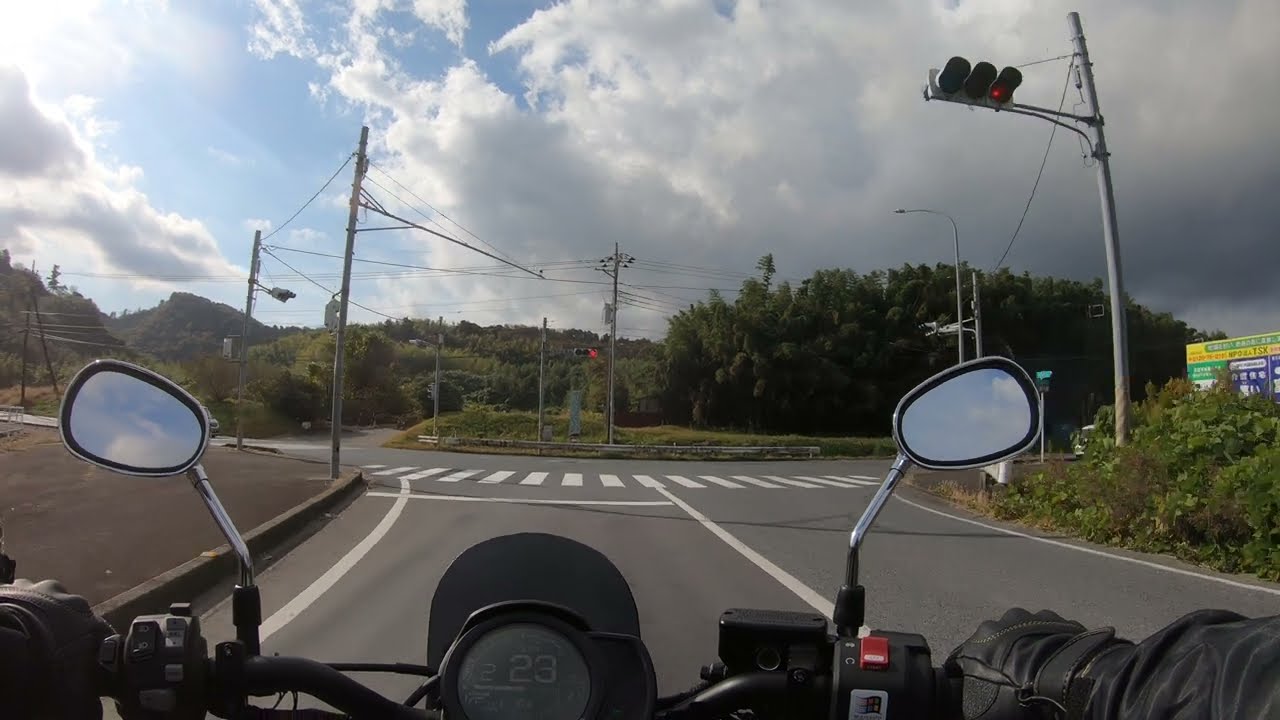In this daytime photograph, the viewer is given a perspective from a camera likely chest-mounted on a motorcyclist. The scene shows the front half of a motorcycle, including the handlebars, tachometer reading 23, and two large silver mirrors mounted on silver posts, reflecting the sky. The motorcyclist, wearing black gloves and a black jacket, is in the left lane of a two-lane road, halted at a red traffic light. The intersection ahead hints at multiple directions, possibly a cross street or a roundabout, flanked by a crosswalk. To the right, there is an indistinguishable large sign or billboard. Evergreen trees and green shrubs line the road and extend into the background. Overhead, there's a mix of a blue sky and large, dark clouds, with sunshine illuminating the left part of the image. Overhead wires run across the intersection, and to the left side of the road, a raised concrete area resembles either a parking lot or a non-vehicular zone.